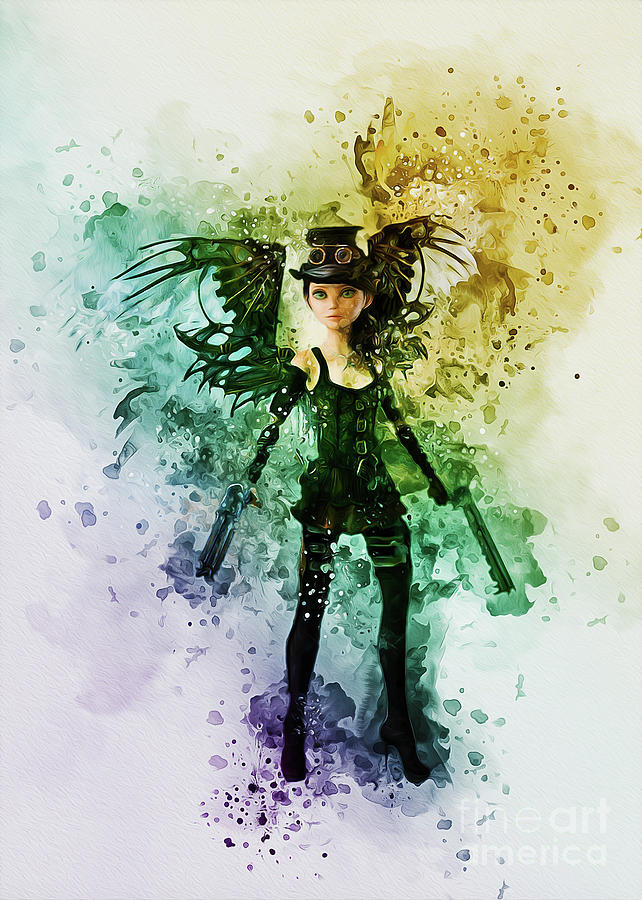The image is a highly stylized digital painting blending fantasy and sci-fi elements. It features a teenage girl in a steampunk-inspired outfit, prominently situated against a dreamy, watercolor-like backdrop. She wears a leather corset accentuated with brass buckles and a short black skirt. Her thigh-high black boots with high heels extend up to just beneath the skirt, and she's adorned with long black gloves. Her piercing green eyes stand out, and atop her head is a steampunk-style top hat with a visor reminiscent of something from a Jules Verne novel. This hat is adorned with goggles, adding a touch that evokes the style of Slash from Guns N' Roses. Her wings are a striking combination of black feathers and mechanical elements, resembling a fusion of bat wings and machinery. In one hand, she clutches a sawed-off shotgun, while the other arm appears to be a weapon itself, perhaps robotic. The background swirls with psychedelic colors, including gold in the upper right, green on the left, and purple beneath her feet, creating a misty, ethereal aura around the character. The painting masterfully uses brush strokes that splatter outwards, enhancing the fantasy-meets-sci-fi aesthetic.